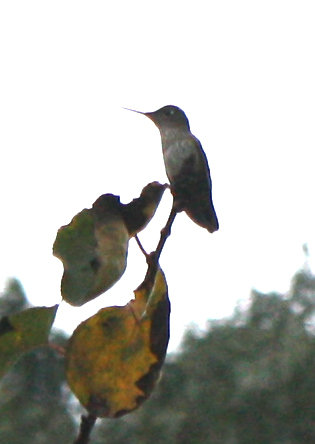In this image, a small hummingbird is perched delicately on the tip of a branch, surrounded by three withered leaves that are predominantly orange, brown, and gray in color. The bird, facing left, is distinguished by its characteristically slender beak and small head. Its head and tail feature darker feathers, while a prominent white ring encircles its neck, extending from the back of its head to the front of its chest. Behind the bird stretches an out-of-focus collection of trees set against an overcast, white sky, creating a muted ambiance that slightly obscures the bird’s full coloration. The overall setting is outdoors, captured in soft lighting that highlights the tranquil scene.